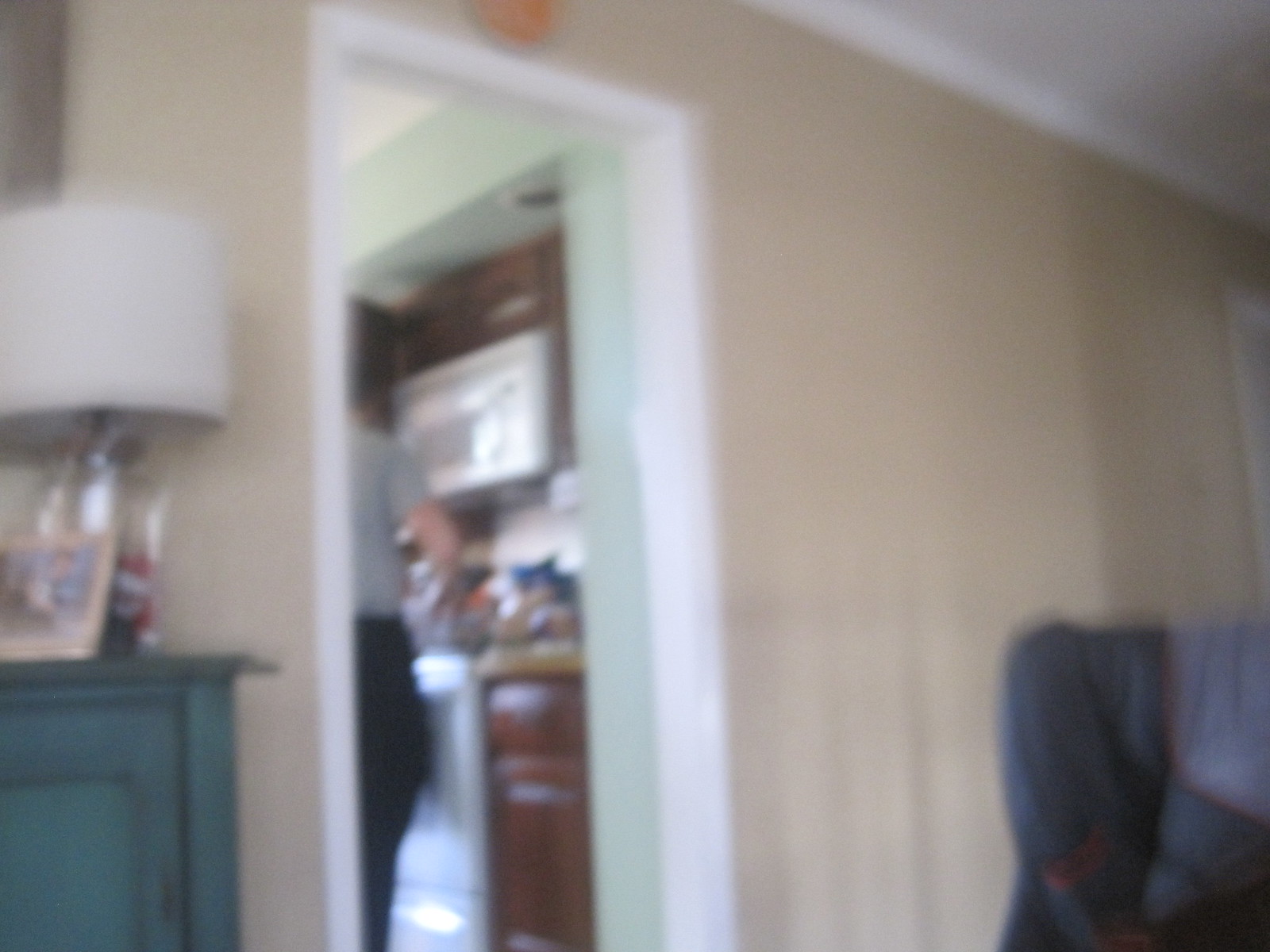The image depicts a dimly lit room adjacent to a kitchen, viewed through an open, white-framed doorway on the left side. The room's walls are a light brown or tan color. Inside the doorway, a blurry figure stands in the kitchen, wearing a short-sleeved gray T-shirt, black pants, and having short brown hair. He appears to be using a range stove, with his arm engaged in some cooking activity. Above the range, a white microwave is built into the dark wooden cabinets, possibly oak or dark cherry. Some bags of food clutter the countertops alongside the microwave. The kitchen ceiling features recessed lighting with two can lights.

To the left of the doorway in the adjacent room stands a dark green or blue wooden cabinet. Atop this cabinet is a lamp with a beige, cylinder-shaped lampshade and a clear base. Additionally, there is a picture frame with a light brown wooden border, seemingly displaying a photo, though the image is too blurry for details. On the right side of the image, part of a TV covered with a blanket and some shadowing are visible, adding to the contrast between the dimly lit adjacent room and the brighter kitchen interior. Moreover, near the top of the kitchen doorway, a round, red object that resembles a fire alarm can be seen. Draped over a chair on the bottom right corner of the image is a fabric resembling a jacket with red line designs, further emphasizing the lived-in feel of the space.